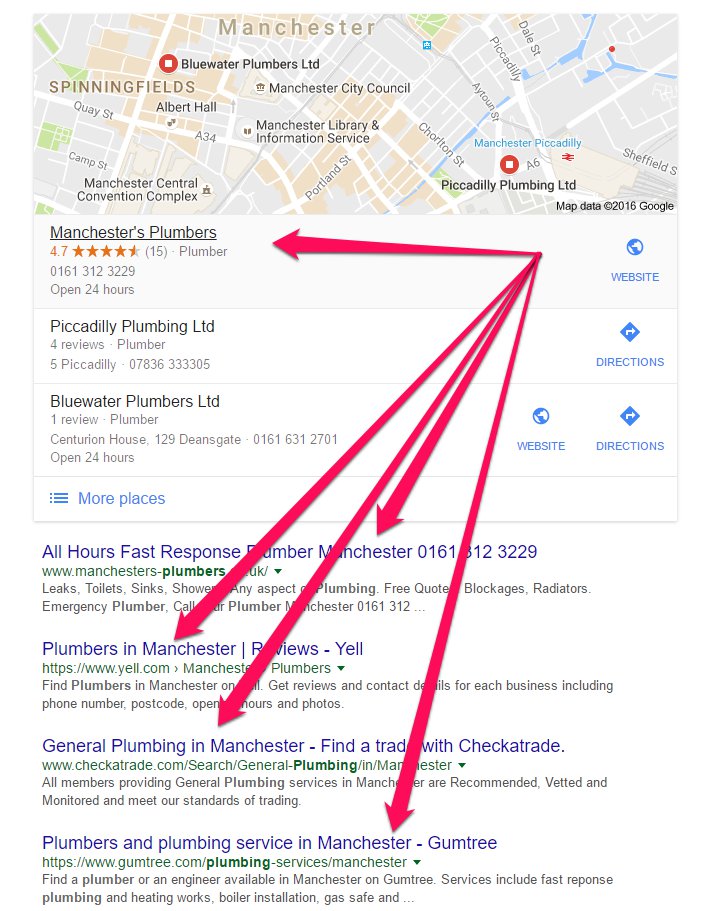This image captures a Google search results page focusing on plumbing services in Manchester, United Kingdom. At the top of the page, there is a city map highlighting Manchester and Springfield areas, showcasing various local businesses related to plumbing services.

Below the map, three plumbing businesses are listed with detailed information:
1. **Masters Plumbers**
   - Rating: 4.7 stars from 15 reviews.
   - Contact: Phone number provided.
   - Availability: Open 24 hours.
   - Website: Accessible via a blue icon and text indicating the presence of a website.

2. **Piccadilly Plumbing Ltd.**
   - Rating: 4 stars from 4 reviews.
   - Contact: Phone number and address provided.
   - Additional Feature: Directions button available.

3. **Blue Water Plumbers Ltd.**
   - Rating: 1 star from 1 review.
   - Contact: Phone number and address provided.
   - Availability: Open 24 hours.
   - Additional Features: Website accessible via icon and text; directions available.

Below these business listings, there are four related links:
- "All hours fast response plumber Manchester"
- "Plumbers in Manchester reviews from Yell"
- "General plumbing in Manchester from Checkatrade"
- "Plumbers and plumbing services in Manchester from Gumtree"

A red arrow is pointing towards specific businesses and links, possibly indicating highlighted or sponsored results.